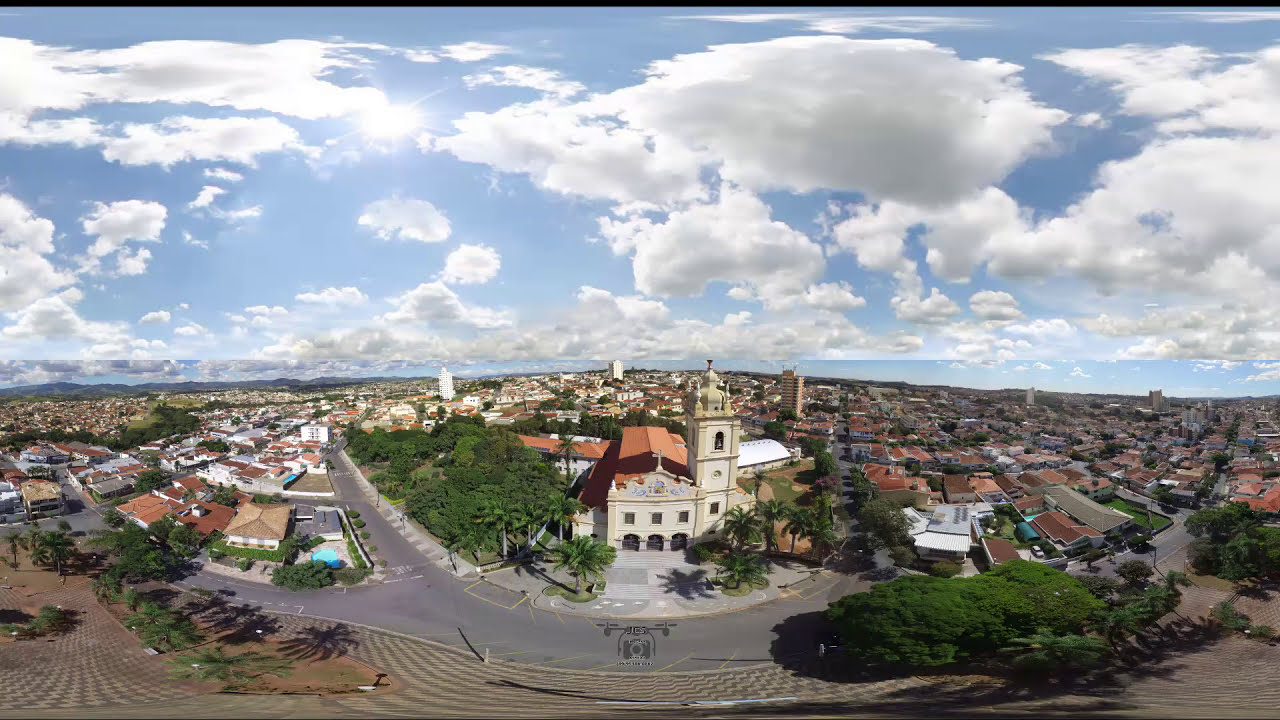This image is a rectangular aerial photograph capturing a picturesque European town on a bright, sunny day. The viewpoint is from high above, possibly from a plane or a helicopter, offering a bird’s-eye view that stretches for miles. The town is predominantly residential, characterized by an array of buildings with brownish-reddish terracotta roofs and walls in shades of brown and white. The tallest structure is a church with a prominent steeple situated at the center, at the junction of two streets. 

In the immediate foreground, a brown plowed field and a road are visible, beyond which the town begins. Trees and shrubs, along with some green spaces, are interspersed among the buildings, casting long shadows on the gray streets. Notably, there are archways at the forefront of the main visible building and a building with a swimming pool across from the church to the left with a small grove of green trees nearby. 

The upper half of the image is dominated by a beautiful sky, where the sun peeks out from behind fluffy, white cumulus clouds, some tinged with gray. The distant horizon blends into the sky’s expanse, creating a serene backdrop. Despite the town’s apparent bustle, no people are visible due to the high vantage point of the photograph. The overall impression is of a quaint, tranquil town bathed in sunlight with a stunning mix of architectural and natural beauty.